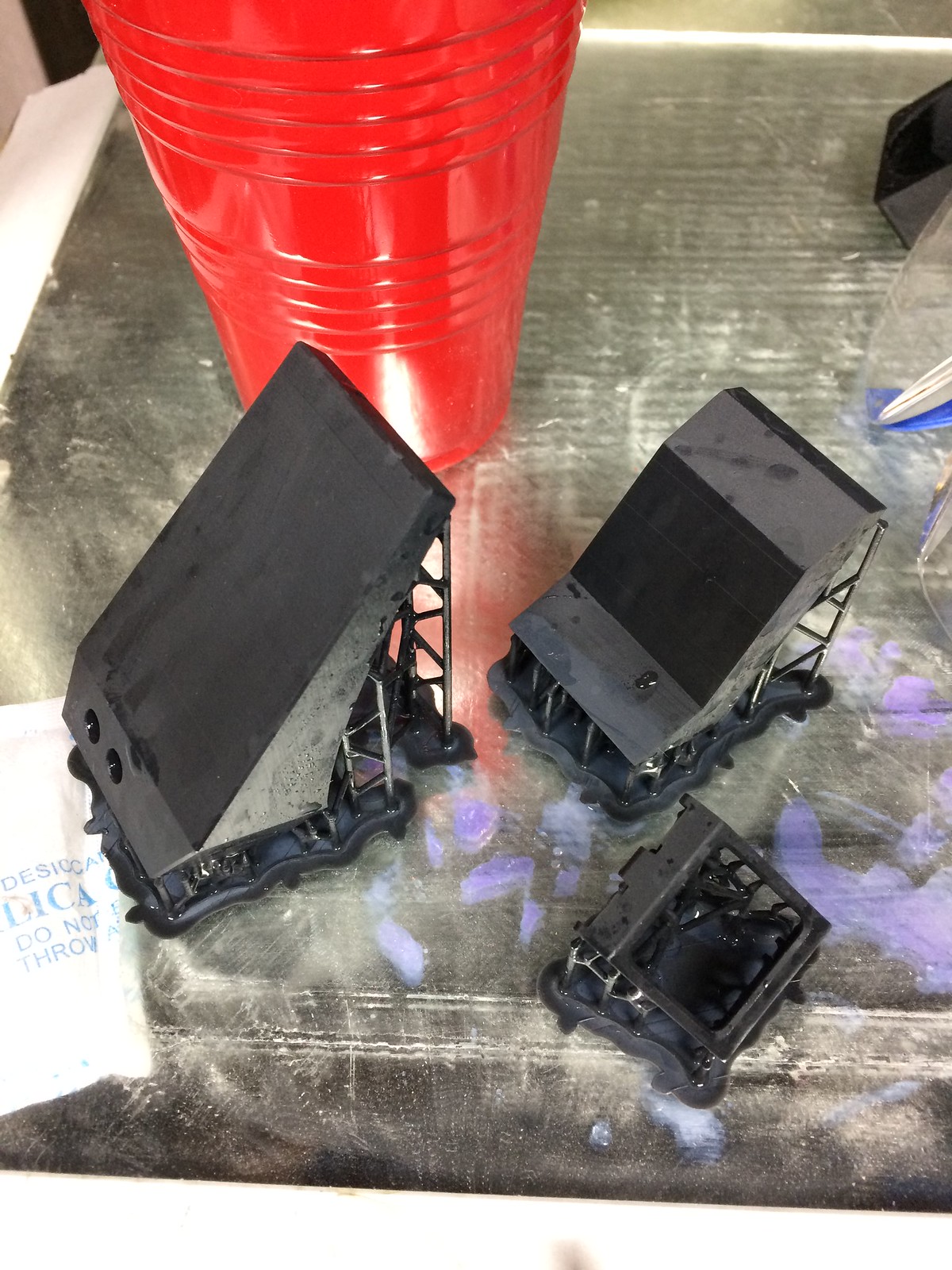The photo captures a cluttered tabletop with a reflective glass or mirror surface, smudged and speckled with a white substance. Prominently, there is a bright red solo cup situated in the upper left corner. Nearby, three miniature black structures, likely 3D-printed ramps or parts of a scale model, are arranged. These structures vary in design: one is steep, another features multiple bends, and the third has a hole. In the lower left of the image lies a white silica gel packet with blue text warning "Do Not Eat." Scattered around these items are purple splatters, adding to the tabletop’s chaotic appearance.